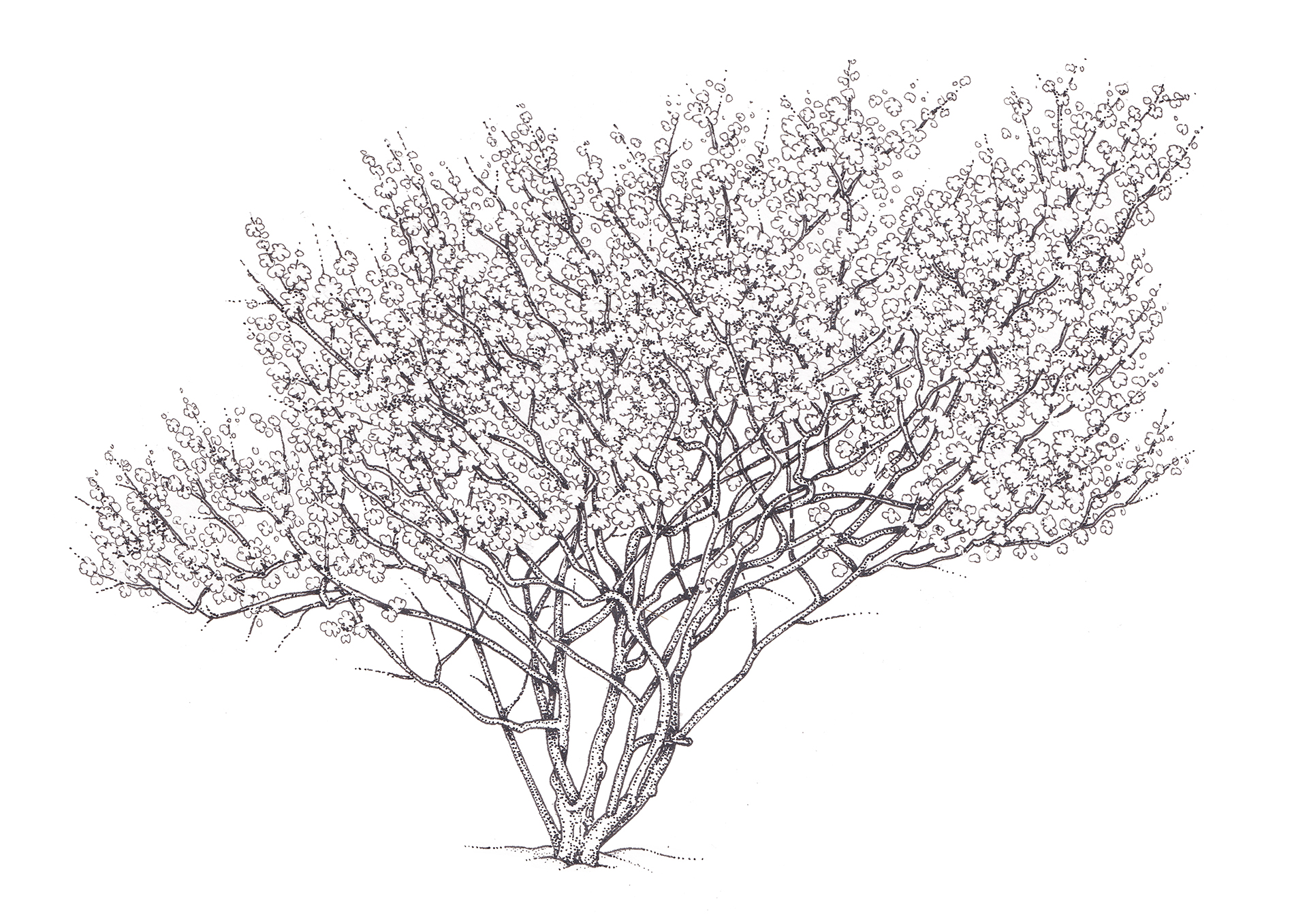The image is a detailed black and white pencil drawing of a tree that resembles a bush, with all branches expanding outward from a short base that emerges directly from the ground. The tree features numerous small, cloud-like leaves or flowers clustered densely on its many branches, creating a large, fluffy canopy. The backdrop is entirely white, emphasizing the intricate details of the tree. The base of the tree is grounded in what appears to be a dirt area, suggested by the slight marks on the ground around it. Despite the lack of color, the textures and forms are finely depicted, making the tree appear as if it is in full bloom, typical of a spring scene.